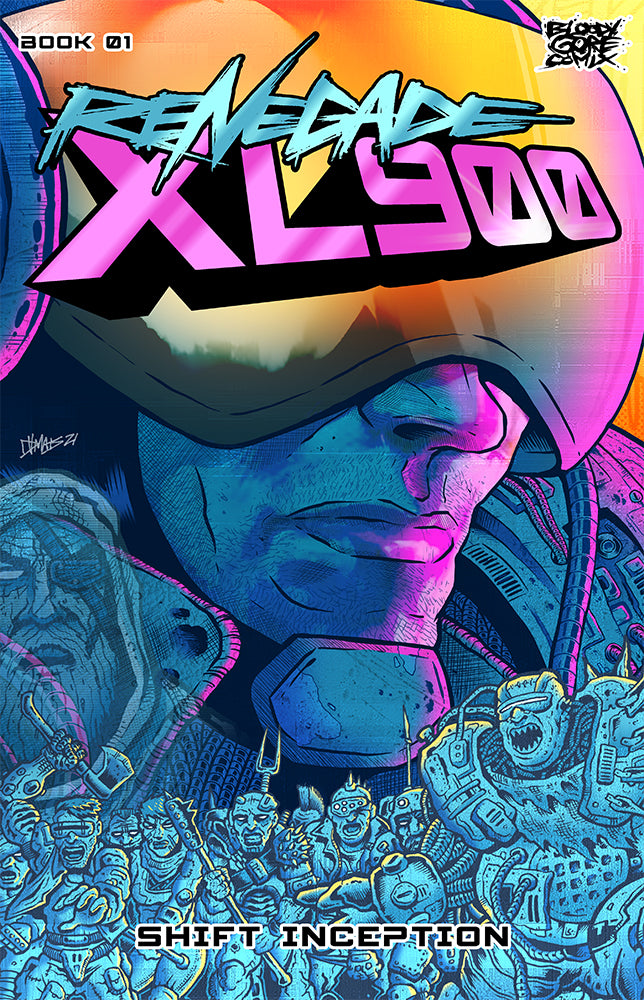The cover of the comic book "Renegade XL900" prominently features a large, reflective orange helmet worn by a man, partially obscuring the upper part of his face. A futuristic pink light shines across his face, adding a sci-fi tone to the bluish-tinted visage. Above the man's head, the title "Renegade" is written in a light blue, sketchy, hand-drawn font, with "XL900" below it in a bold, futuristic block font. In the upper left corner, "Book 01" is displayed in black letters with a white outline, while the upper right corner features the publisher's name, "Bloody Gore COMIX," also in black with a white outline. Below the man's face, an ominous assembly of heavily armored, Mad Max-style warriors are depicted carrying pitchforks, bathed in a blue tint. The title "Shift Inception" is written in black text at the bottom, suggesting an epic battle against this horde of monstrous figures.